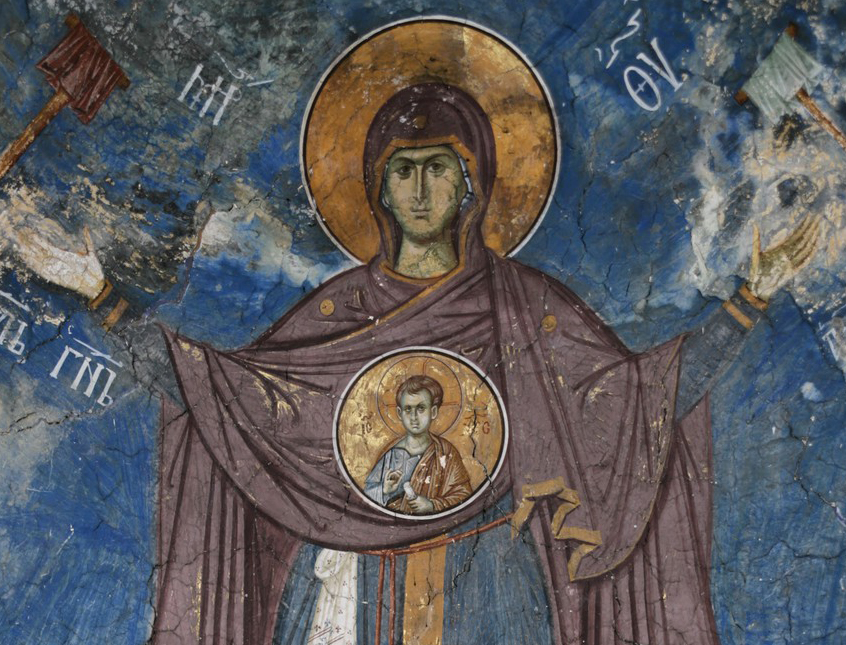The image depicts an ancient, damaged painting on a domed ceiling, showcasing a saint or the Madonna with a gold halo. The figure stands with arms outstretched, adorned in a layered ensemble featuring a blue gown with strings at the waist and a purple robe. A scarf veils the head, with the face clearly visible. Draped across the shoulders and extending possibly to the floor is a cloth. Central to the chest is a medallion with a smaller figure, likely depicting the child Jesus, who is haloed and holds a rolled document in one hand, making a holy gesture with the other. Surrounding the main figure is Cyrillic writing, set against a backdrop of blue that might represent the world.